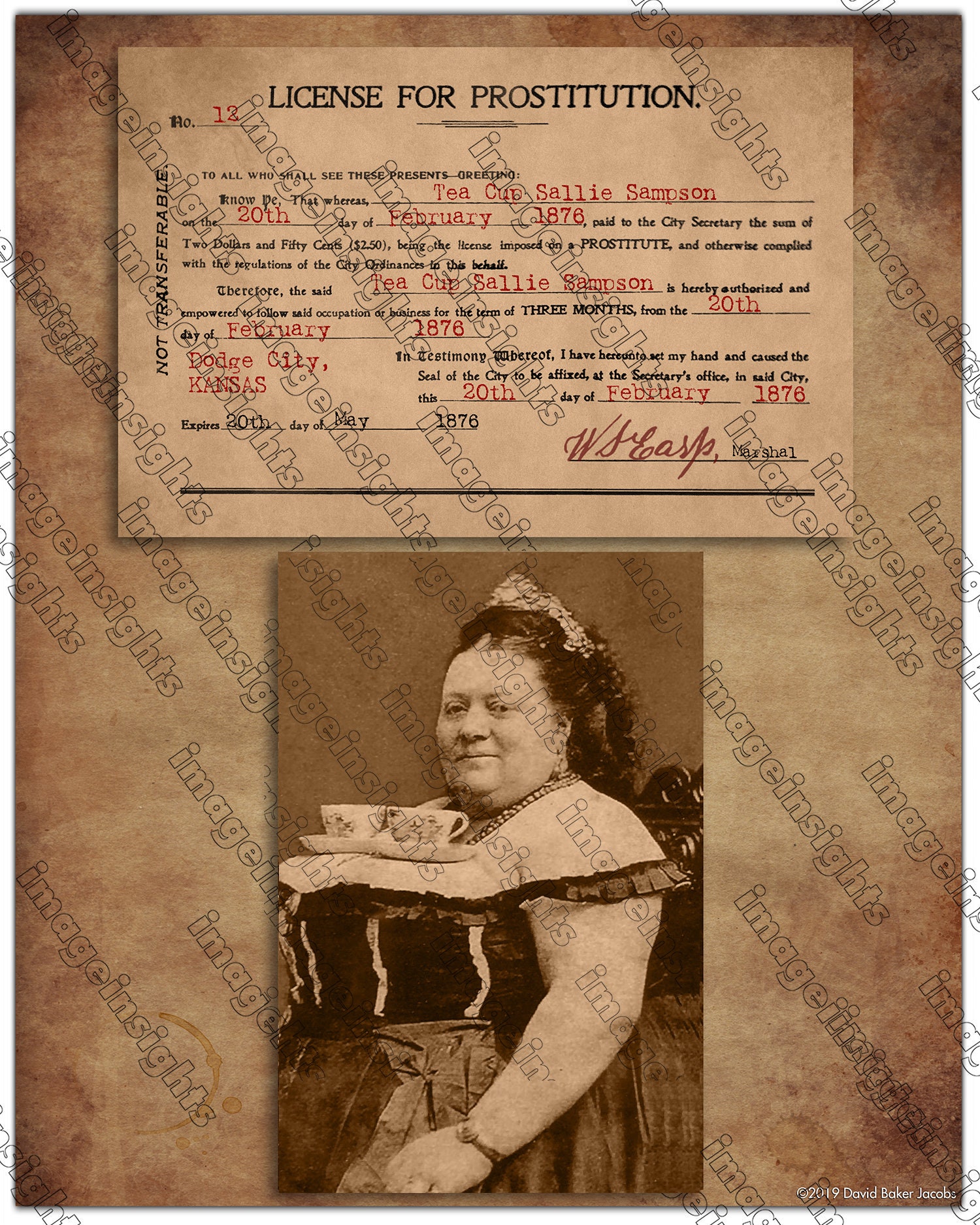This vintage photograph, in sepia tones, portrays a larger woman identified as Teacup Sally Sampson, taken on February 20th, 1876. She is seated with elaborate hair and a fancy dress, accentuated by a corset top and a skirting. She is balancing two teacups and saucers on her chest, and she wears a bracelet on her wrist. Positioned above her image is an official-looking document titled "License for Prostitution, number 12," certifying her as a licensed prostitute in Dodge City, Kansas. The document features black text with blank spaces filled in with red typewritten information, adding authenticity to this historical piece.